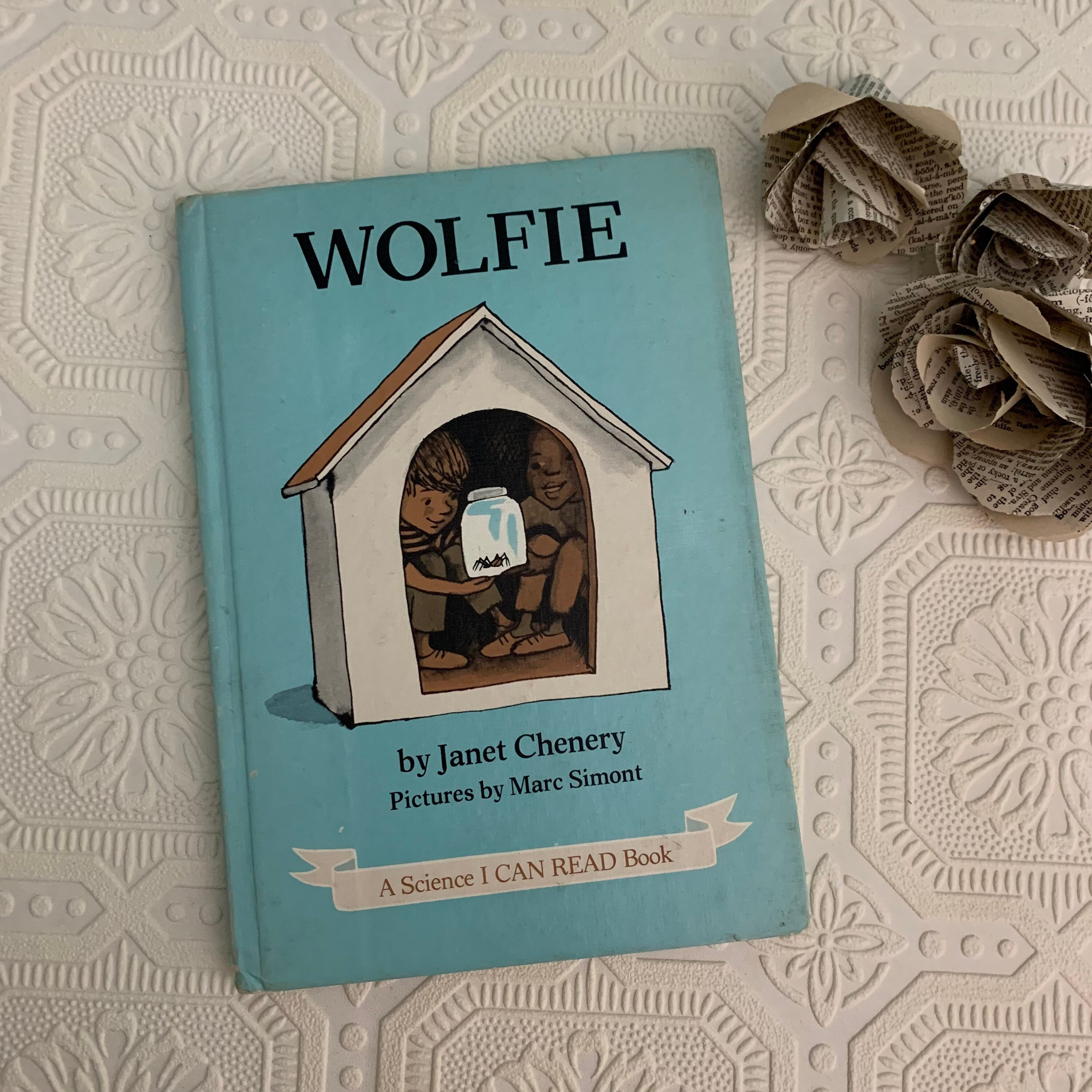This square-shaped photograph features a children's book titled "Wolfie," prominently displayed on a white, intricately textured surface that resembles a tiled floor or table. The elegant background includes a pattern of repeating squares and flowers, adding a sophisticated touch. In the upper right corner, two flowers crafted from newspaper stand out, with the larger one situated closer to the center of the image.

The book itself has a Tiffany blue cover that appears slightly weathered, giving it a vintage charm. "WOLFIE" is printed in bold black capital letters at the top. Below the title, a white doghouse with an orange roof is depicted, sheltering two smiling children who are holding a jar containing a large black spider, possibly Wolfie. At the bottom of the cover, "By Janet Chenery," and "Pictures by Mark Simont" are written in black text. A white ribbon at the very bottom of the cover displays the phrase "A Science I Can Read Book" in red font.